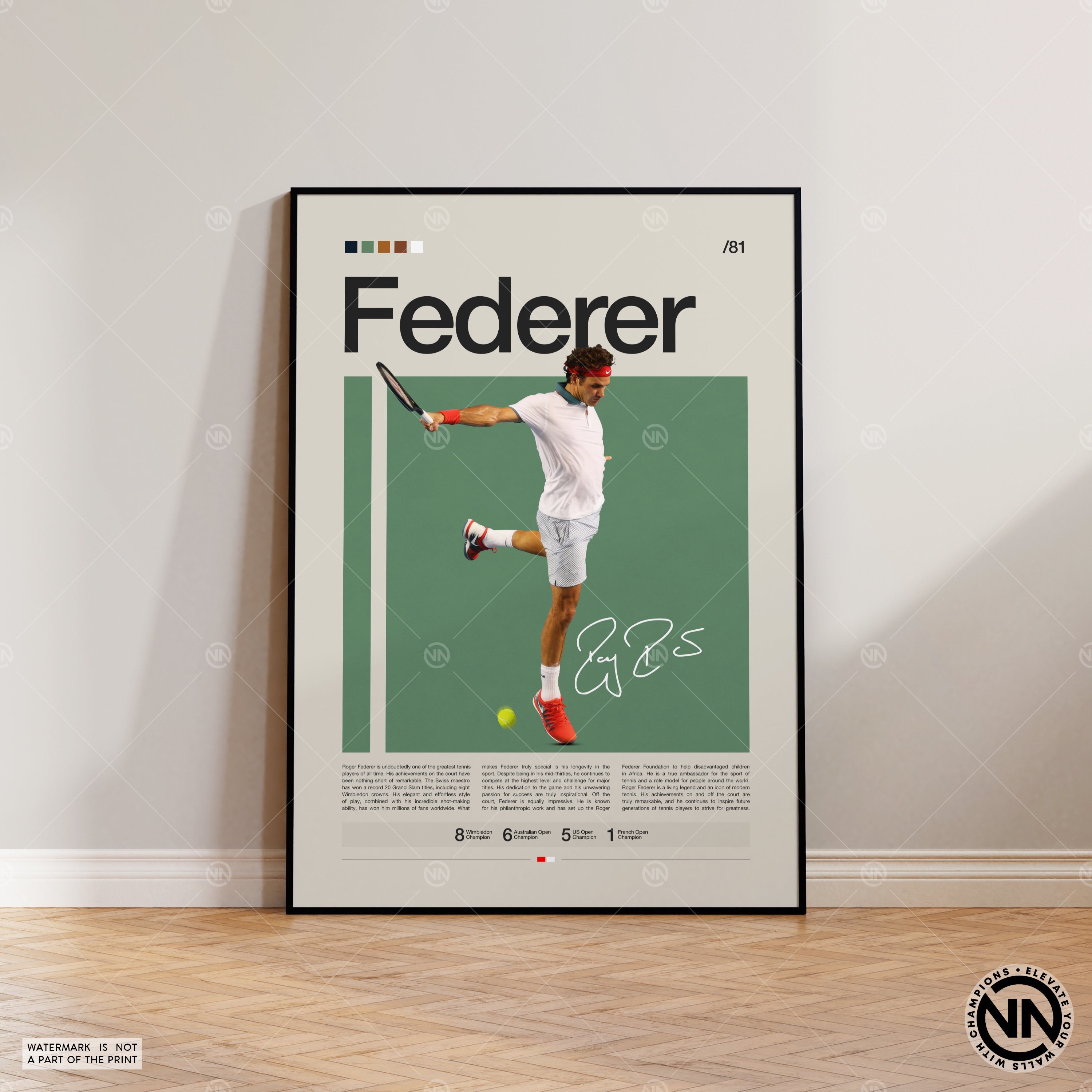The image depicts a large framed picture leaning against a light gray or off-white wall, with a wood-patterned floor beneath it. The frame has a thin black border and inside, the background of the picture is also gray. At the top of the framed picture, bold black letters spell out "FEDERER". Below the text, there is a green square that highlights an image of a tennis player, identified as Roger Federer, standing on one leg with his right arm extended, holding a racket. The player is dressed in a white shirt and gray shorts, complemented by orange wristbands, orange shoes, and white socks. A tennis ball is seen bouncing on the ground near the player's foot. The picture also features a signature to the right of Federer's leg and a logo in the bottom right corner that reads, "Elevate your walls with champions". The floor has a textured zigzag pattern in light and dark brown shades. Additionally, there is a small rectangle at the bottom left of the picture that states, "watermark is not a part of the paint". The frame also includes subtle watermarks, described as light white diamonds with the symbol "NN" at the intersections. At the bottom of the frame, illegible text is followed by the numbers "8651" with additional text extending from each digit.